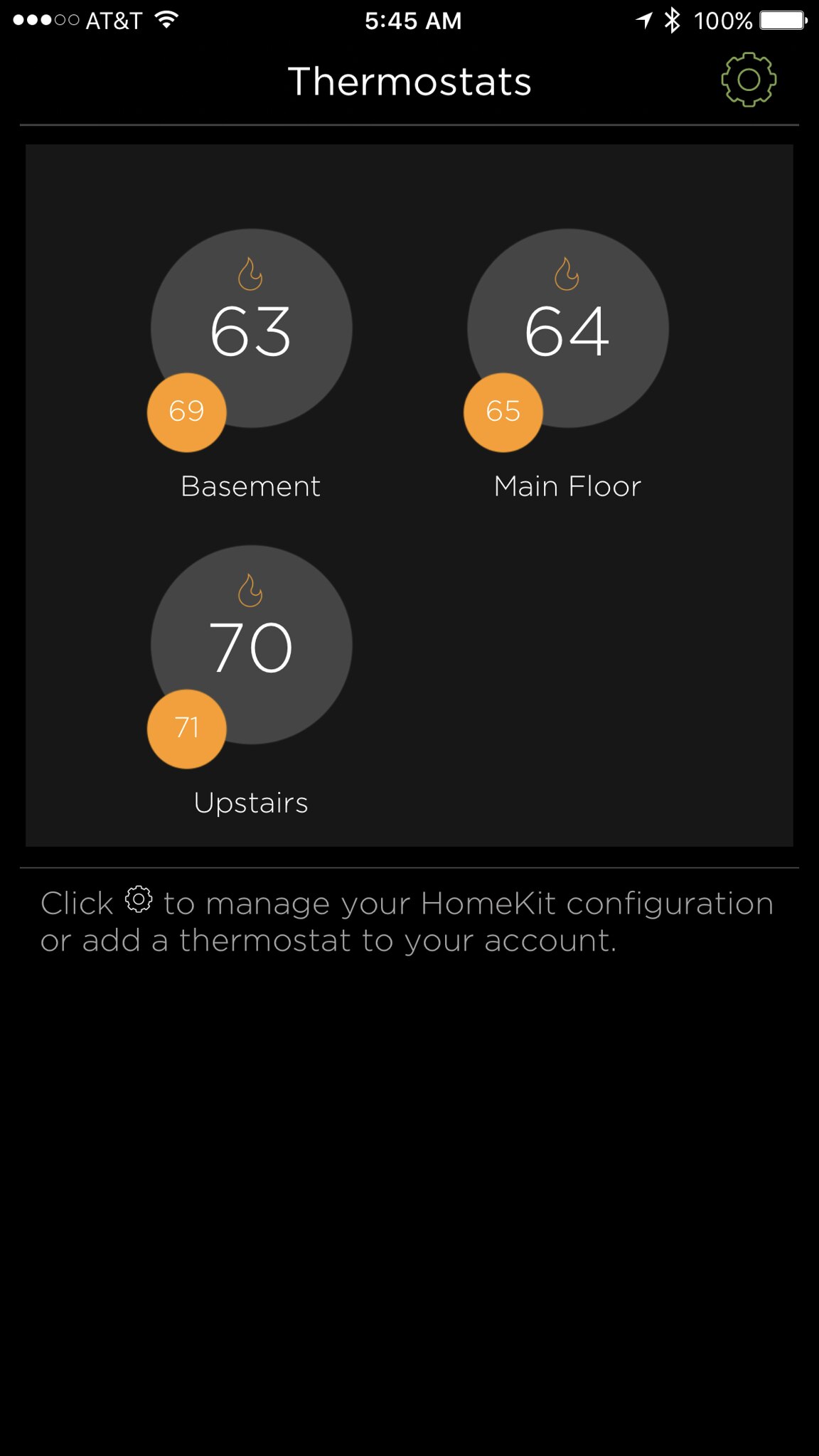A screenshot of a smart thermostat app interface in dark mode. 

At the top of the screen, there are various status icons: three out of five signal bars for AT&T, a Wi-Fi signal icon, the time displayed as 5:45 a.m., a location icon, a Bluetooth icon, and a battery icon showing 100% charge—all in white.

Below this, the screen title "Thermostats" is displayed alongside a settings wheel icon. The background is black, suggesting dark mode is enabled.

The main section of the interface shows three circles indicating temperature readings for different areas of the home. The first circle reads "63°F" labeled "Basement," and the second circle reads "64°F" labeled "Main Floor." Both circles have a small orange indicator in the bottom left corner.

Below these, a larger gray circle displays "70°F" with a small orange indicator reading "71°F" labeled "Upstairs."

At the bottom of the screen, a message in white text instructs users: "Click the settings icon to manage your HomeKit configuration or add a thermostat to your account."

The entire interface is set against a dark black background, providing a clear contrast with the white text and icons.